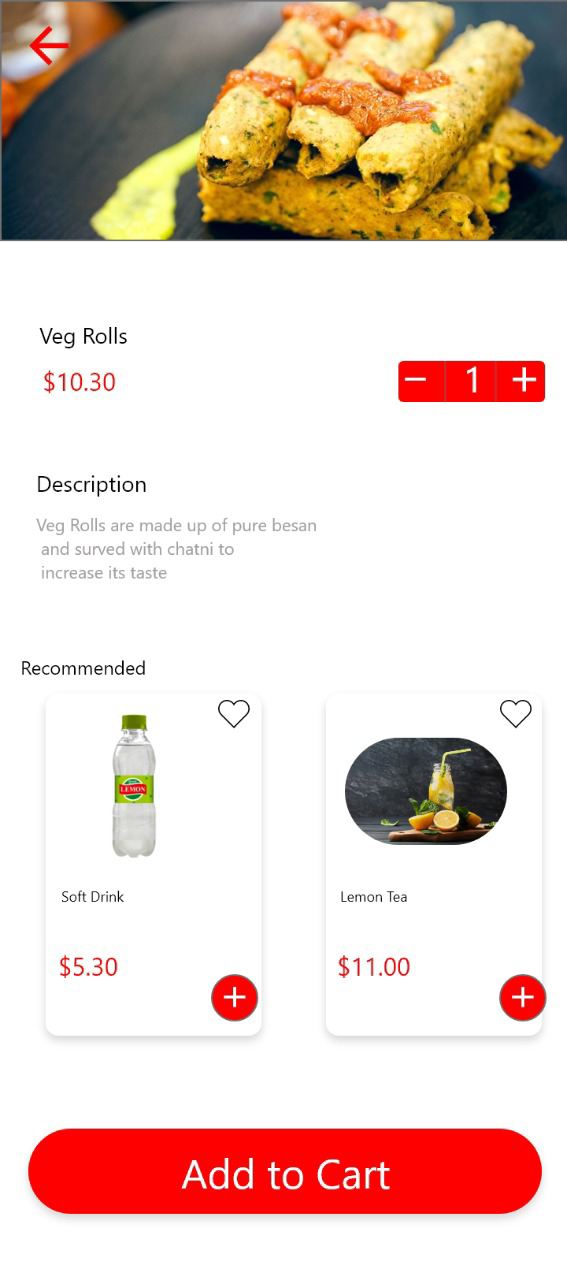The image displays a menu item from a website, showcasing a dish titled "Veg Rolls". At the top of the image, there is a picture of the dish, featuring six yellowish rolls arranged in a crisscross pattern on a black plate. The top three rolls have a red sauce drizzled over them. Below the image, the item's price is listed as $10.30. 

To the right of the price, there's a quantity selector consisting of a red minus button, a 1 in the center, and a red plus button. The item's description reads: "Veg rolls are made up of pure besan and served with chutney to enhance their taste."

In the upper-left corner of the image, there is a red arrow pointing back. Beneath the main item, the section shows a couple of recommended items: a soft drink priced at $5.30, and lemon tea priced at $11. Both recommendations have a red plus icon at their bottom right corners for easy addition to the cart, and a heart icon in the top right for adding to favorites.

At the bottom of the display, there's a prominent red button labeled "Add to Cart."